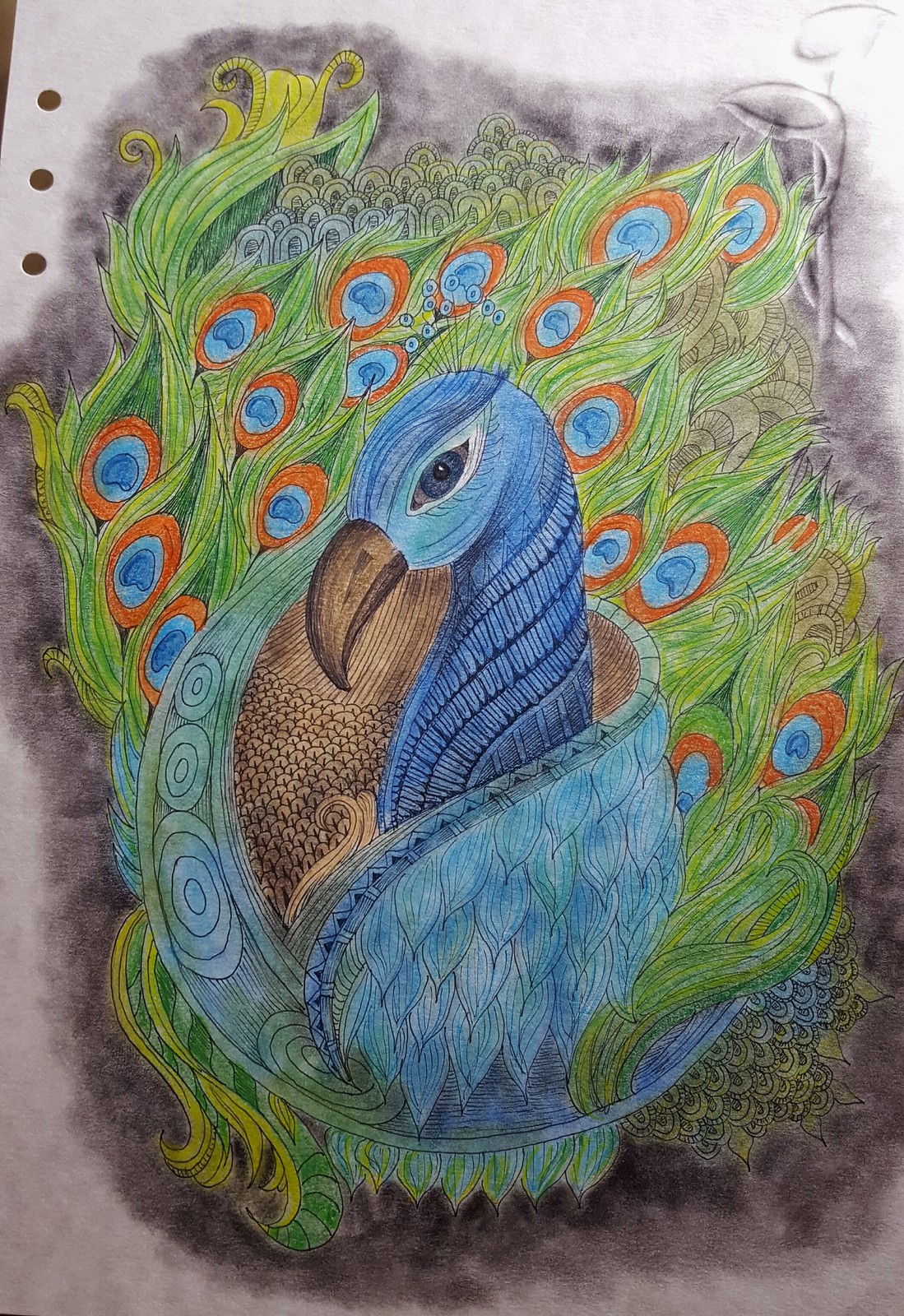This vibrant mixed media illustration of a peacock is detailed on sketch paper with three punched-out holes along the top left corner, suggesting it was removed from a notebook. The peacock, drawn with a combination of colored pencils and possibly pen or watercolor, is shown in profile, sitting with its head turned towards the left. Its striking blue head, adorned with blue circular feathers, features a blue eye and a long, curved brown beak. The neck and chest of the bird exhibit a subtle brown hue with a textured, scaly appearance. The wings, wrapped gracefully around its body, are predominantly blue. The magnificent tail feathers, fanned out behind, are green with distinctive eye decorations. These eyes are primarily blue but feature intricate details, including an orange or red outer ring. The illustration captures the peacock's regal posture and dazzling plumage, making it clear that this is a male peacock, renowned for its brilliant, colorful display.